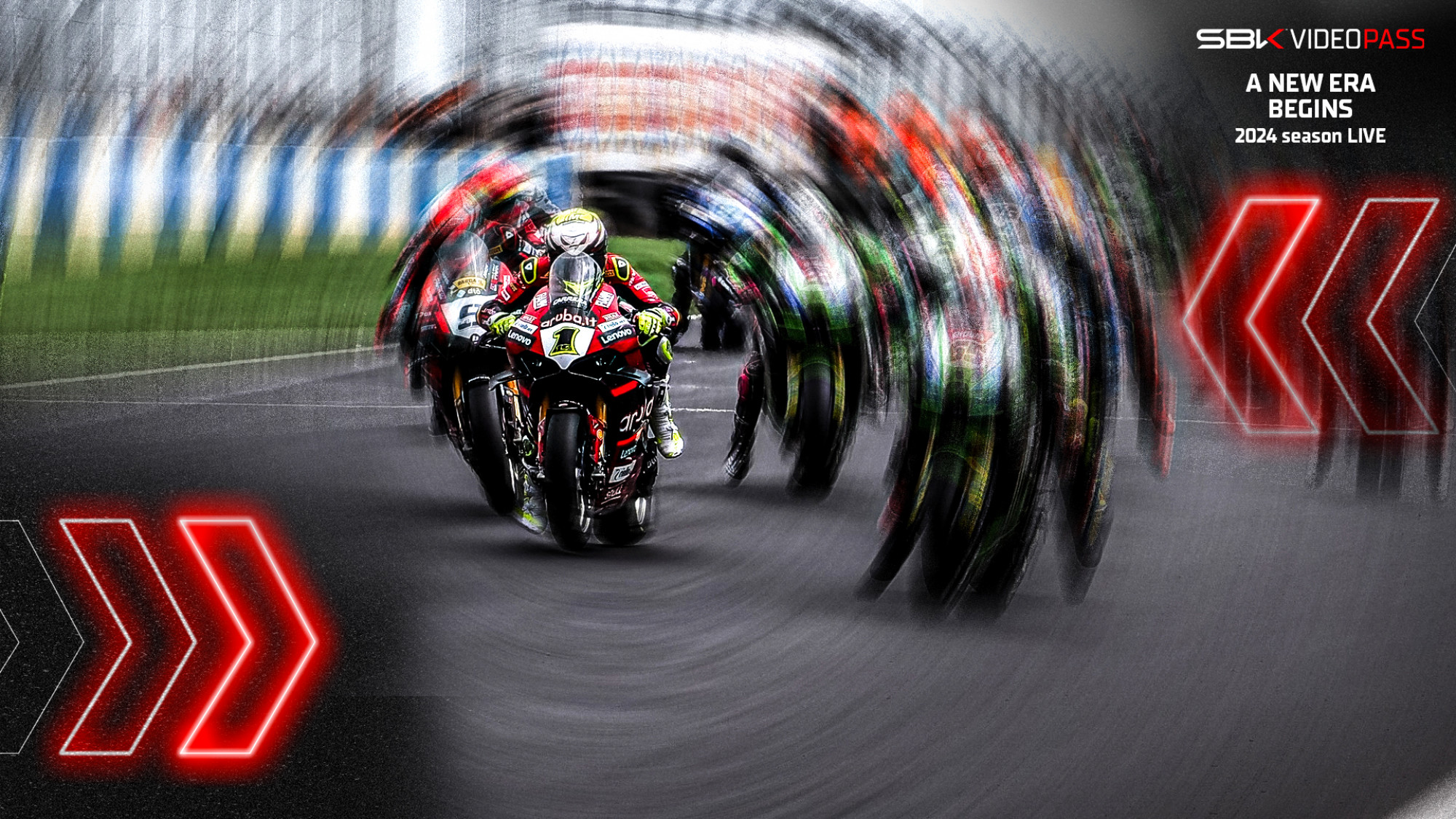This is a heavily edited, full-color photograph of a high-paced motorcycle race captured at track level. The image prominently features one racer in sharp focus, wearing a red and green uniform with a matching red and black motorcycle. Surrounding him, other racers appear blurred in a dynamic circular pattern, creating a "ripple effect" that gives the impression of double vision or motion. The image is horizontally rectangular, adorned with neon red chevron arrows on both sides, adding to the dynamic, futuristic feel. In the top right corner, white text reads "SBK Video Pass, A New Era Begins, 2024 Season Live." The racetrack edge, some grass, and grandstands in blue and white can also be seen, along with a possible advertising signboard, providing context to the scene. The photo's digital enhancements emphasize the sense of speed and competition.